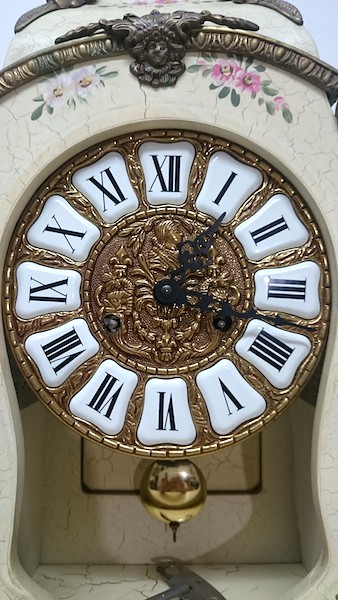This detailed color photograph, in portrait orientation, features an extreme close-up of an ornate analogue clock. The clock's face dominates the image, displaying black Roman numerals housed within small, undulating white tiles that resemble human teeth, with each numeral set in its own distinct tile. The clock's circular face is richly embellished, primarily gold in color with intricate designs, evoking a sense of European elegance. 

The hour and minute hands are crafted in an ornate wrought black iron style, with each hand artistically shaped to resemble leaves with stems. Beneath the face of the clock, a cut-out reveals a golden ball, which functions as a pendulum, adding to the clock's antique charm.

Surrounding the face of the clock is a body with a cream white surface, subtly accented with crack designs for a vintage effect. The top part of the clock is adorned with pink and white flowers accompanied by green leaves, contributing to the overall ornate and floral design. Additionally, the clock is nestled within an elaborate structure that hints at a pottery-like appearance, incorporating a slightly floral motif and crowned with a small, yet distinct, black emblem.

Overall, the composition and intricate details of the clock, from its tooth-like numeral tiles to the floral embellishments and golden pendulum, reflect a sophisticated fusion of artistic craftsmanship and functional design.